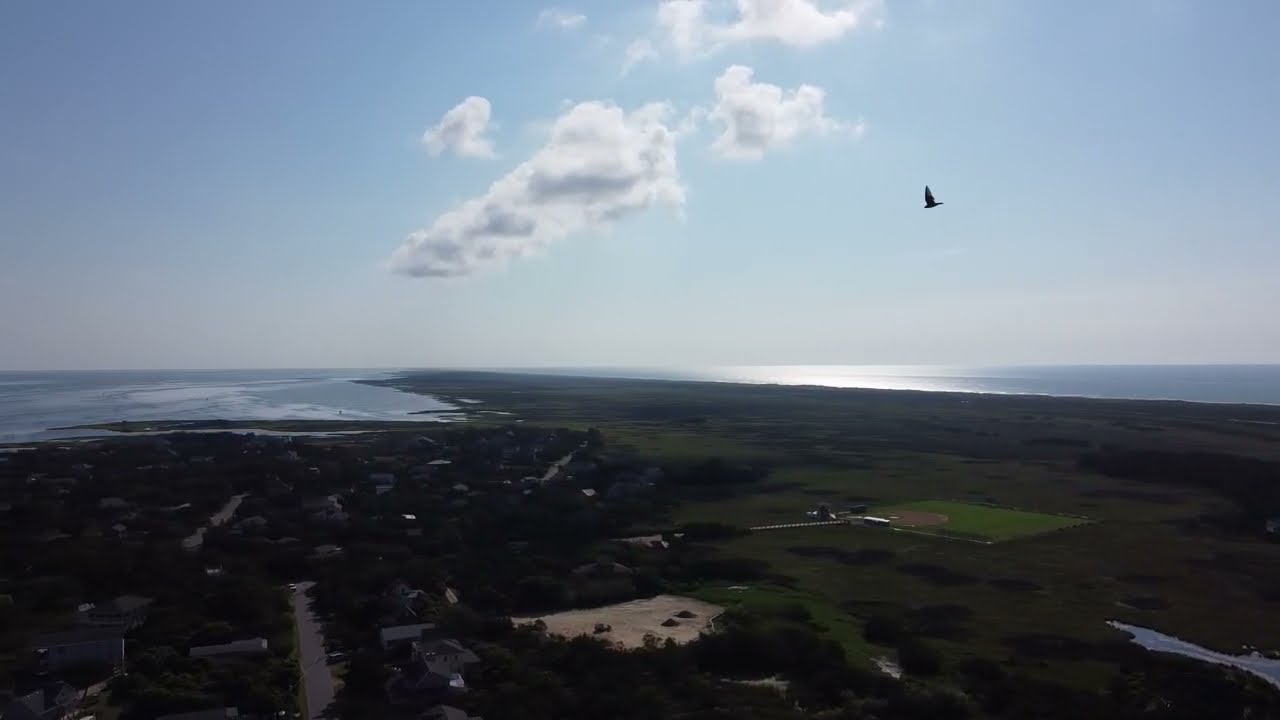This aerial photograph, likely taken from a plane or helicopter, captures a sweeping landscape bathed in daylight. The top half features a vast blue sky with scattered white and gray-bottomed puffy clouds centered in the image. A black bird, possibly an eagle or hawk, soars to the right of these clouds, its solitary wing visible.

Beneath the sky, the land spreads out with intricate details. On the left, a body of water reappears on both sides of the frame, bracketing a wide expanse of lush green foliage. This foliage includes a long peninsula of flat land, peppered with trees, extending towards the horizon where it meets the ocean. The sunlight gently illuminates this peninsula, adding a layer of warmth to the scene.

In the lower left portion, a small town or neighborhood is nestled among a cluster of trees, with visible streets and homes, but devoid of people due to the height of the photograph. Additionally, a large brown, possibly sandy area is evident, along with a baseball field situated in the middle of a treed region. The right edge of the image also reveals a narrow strip of water extending inward. Overall, this detailed overview beautifully combines natural and man-made elements in a serene and picturesque setting.